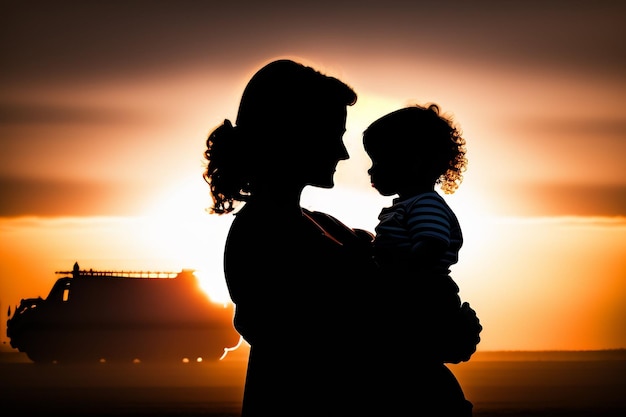The image portrays a captivating scene of a mother and child silhouetted against a breathtaking backdrop of a golden sunset or sunrise. Central to the image, the mother, with her low-hanging hair clip and tightly curled hair, is cradling the child in her arms, both of them locked in an intimate, loving gaze. The child, also with curly hair, is distinguished by a striped shirt, possibly blue or black stripes. The background features a dramatic gradient of colors—from dark gray clouds at the top transitioning into soft pinks, yellows, and oranges, down to a ground of soft yellow fading into dark brown. There is a prominent, shadowy vehicle in the background to the left, possibly a fire engine or mechanical truck with a ladder on top, adding an element of mystery to the serene moment. The overall scene is characterized by its dark hues punctuated with splashes of golden and warm tones, creating a beautifully detailed and evocative image.